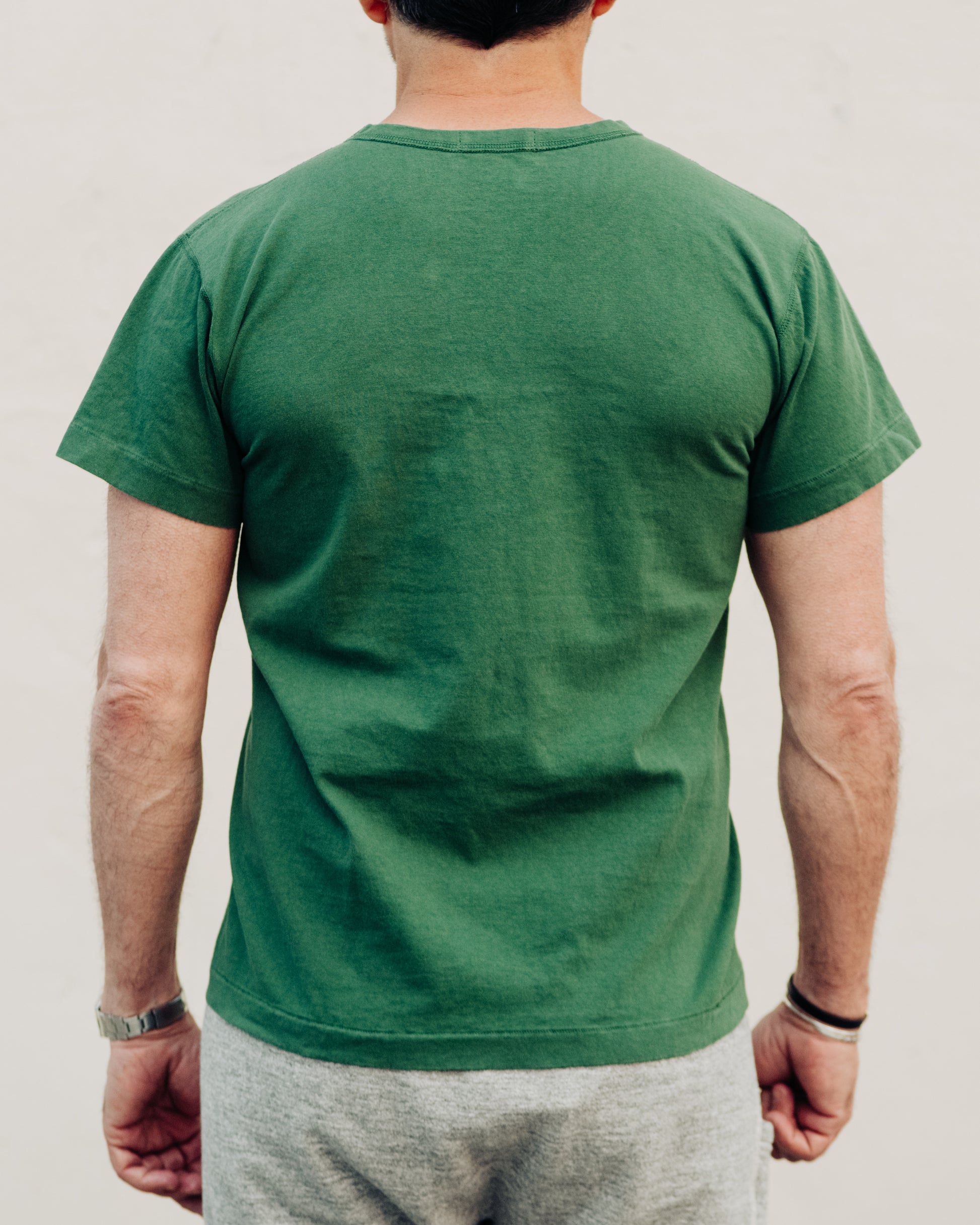In this photograph, we see the backside of an older, muscular White man with short brown hair, cropped from the neck down to his waist. The focus is on his defined back muscles, especially noticeable around the scapula or shoulder area, which stand out prominently. He is wearing a green, short-sleeve t-shirt that appears soft, and gray sweatpants, likely made from a terry cloth material. His forearms reveal veins and hair, emphasizing his fitness. On his left wrist, he wears a silver watch band, and on his right wrist, there are two bracelets, one black and one silver. His hands are clenched, adding to the detailed appearance of his muscular form. The background of the image is a plain white wall, drawing all attention to the man in the center of the frame.